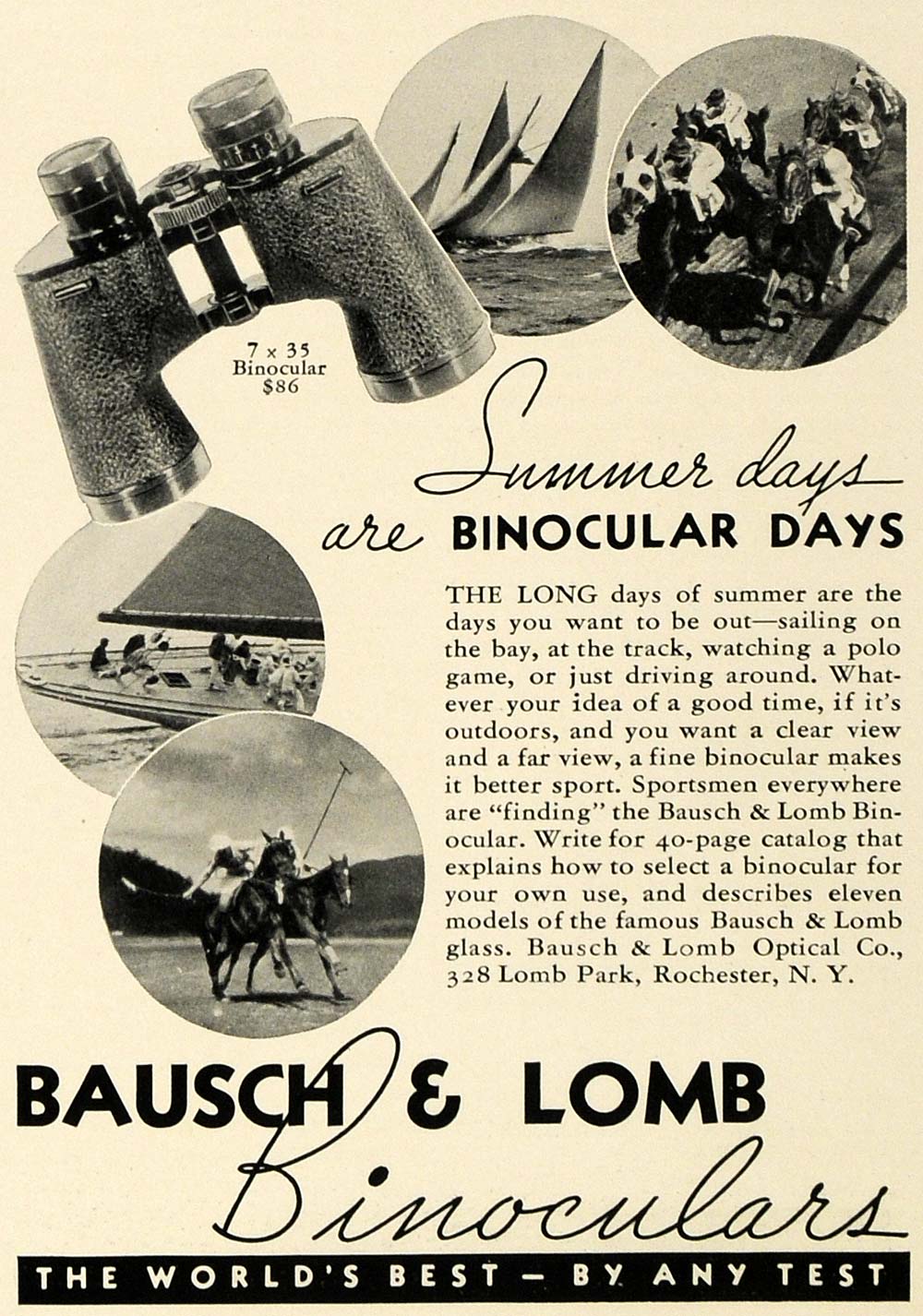This is a scan of an old black-and-white advertisement from a magazine, slightly yellowed with age. The page features a pair of 7x35 binoculars priced at $86 in the upper left-hand corner. Surrounding the binoculars are several grainy circular photographs: one of jockeys racing horses, another of boat sails, a close-up of people on a boat, and an image of someone playing polo on horseback. Beneath these images, a cursive header reads, "Summer days are binocular days." A detailed paragraph below emphasizes the joys of outdoor activities like sailing, horse racing, and polo, suggesting that a good pair of binoculars, specifically the Bausch and Lomb brand, can enhance these experiences. The ad encourages readers to request a 40-page catalog that details how to select binoculars and describes 11 models of the Bausch and Lomb glass. The company's contact information is provided as Bausch and Lomb Optical Co., 328 Lomb Park, Rochester, NY. At the bottom, bold black text reads, "Bausch and Lomb," followed by the tagline, "The world's best by any test."